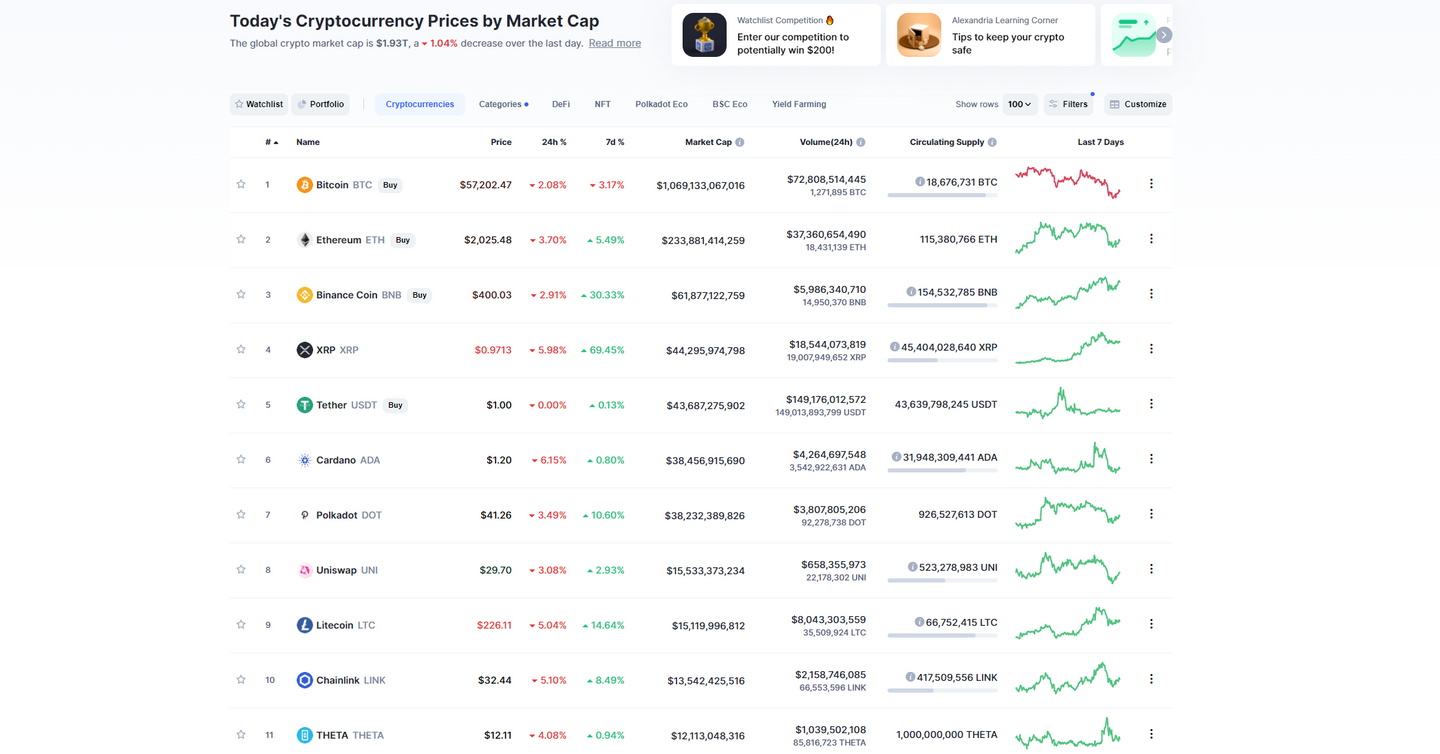In this detailed image, a display of various cryptocurrencies and their current market prices is presented under the title "Today's Cryptocurrency Prices by Market Cap." At the top of the list is Bitcoin (BTC), valued at approximately $57,000. Following Bitcoin is Ethereum (ETH) at $2,025, Binance Coin at $400, and XRP at $0.97. Tether holds steady at $1, while Cardano is priced at $1.20. Polkadot stands at $41.21, Uniswap at $29.70, Litecoin at $226.11, Chainlink at $32.44, and finally, Theta at $12.11. 

The image offers a clear ranking of these cryptocurrencies based on their market capitalization, with Bitcoin leading the chart. The background is primarily white, enhancing readability, and features several menu tabs including options for Watchlist, Portfolio, Cryptocurrency Categories, DeFi, NFT, and Yield Farming. Additionally, the image includes graphs depicting the price trends of each cryptocurrency over the past seven days.